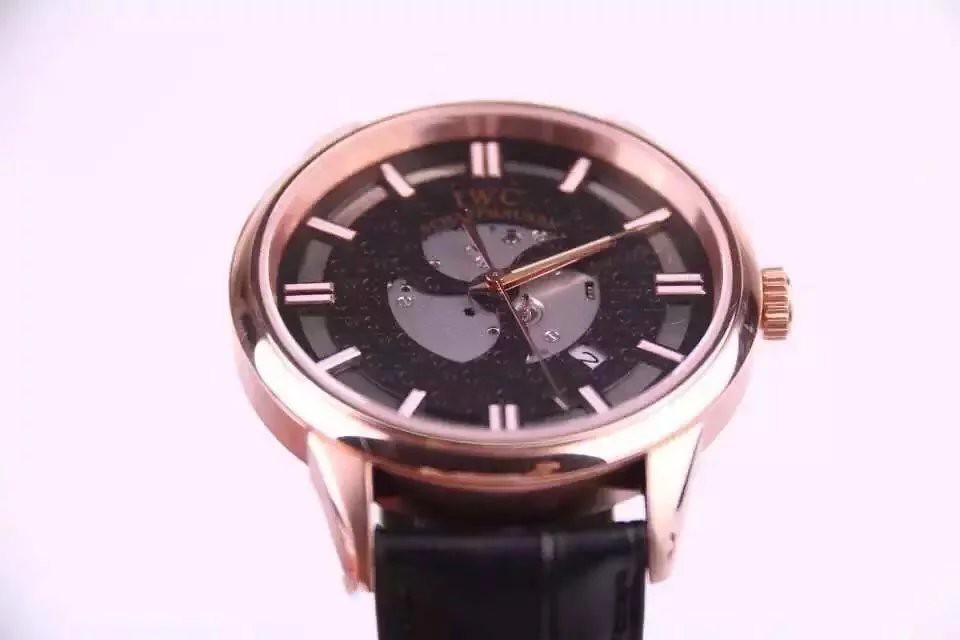This image features a close-up of a gold IWC watch with a black leather strap, set against a bright pale pink background. The watch is slightly tilted, providing a diagonal view of the face. The black dial showcases white markers, with double bars at the 12, 3, 6, and 9 positions, and single bars for the other hours. The time displayed is 11:12, and the date reads the 2nd. Notably, the watch's inner workings are partially visible at the center, adding a touch of intrigue to the sleek design. The watch's crown is situated on the right side of the face, completing its classic look. The pink hue of the background subtly reflects off the golden bezel, adding an elegant ambiance to the scene.